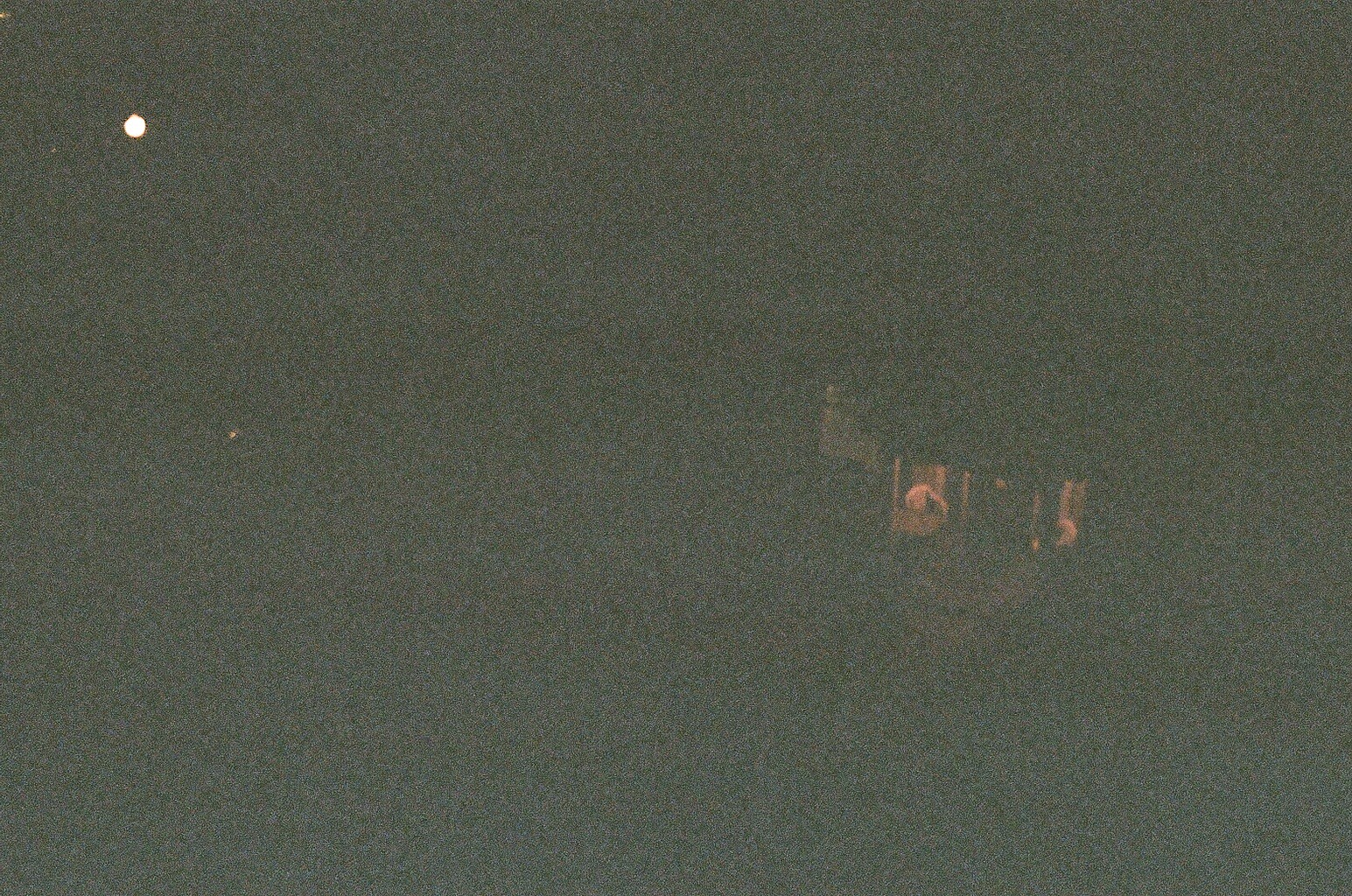This nighttime image is grainy, blurry, and heavily pixelated. Dominating the upper left-hand corner is a prominent white circle, potentially the full moon or a distant light source. Below this, there's a smaller orange dot that might be a star or another type of light. Towards the lower right-center of the image, there's an ambiguous, out-of-focus entity which could be a window or part of a building, giving off a light orange glow. Additionally, patches of red marks and lines can be seen on the right side of the image, hinting vaguely at a shape or structure, although it's too indistinct to identify clearly. The overall dark, grainy, and unfocused nature of the photo makes it challenging to interpret distinct features, leaving much of the scene open to speculation.